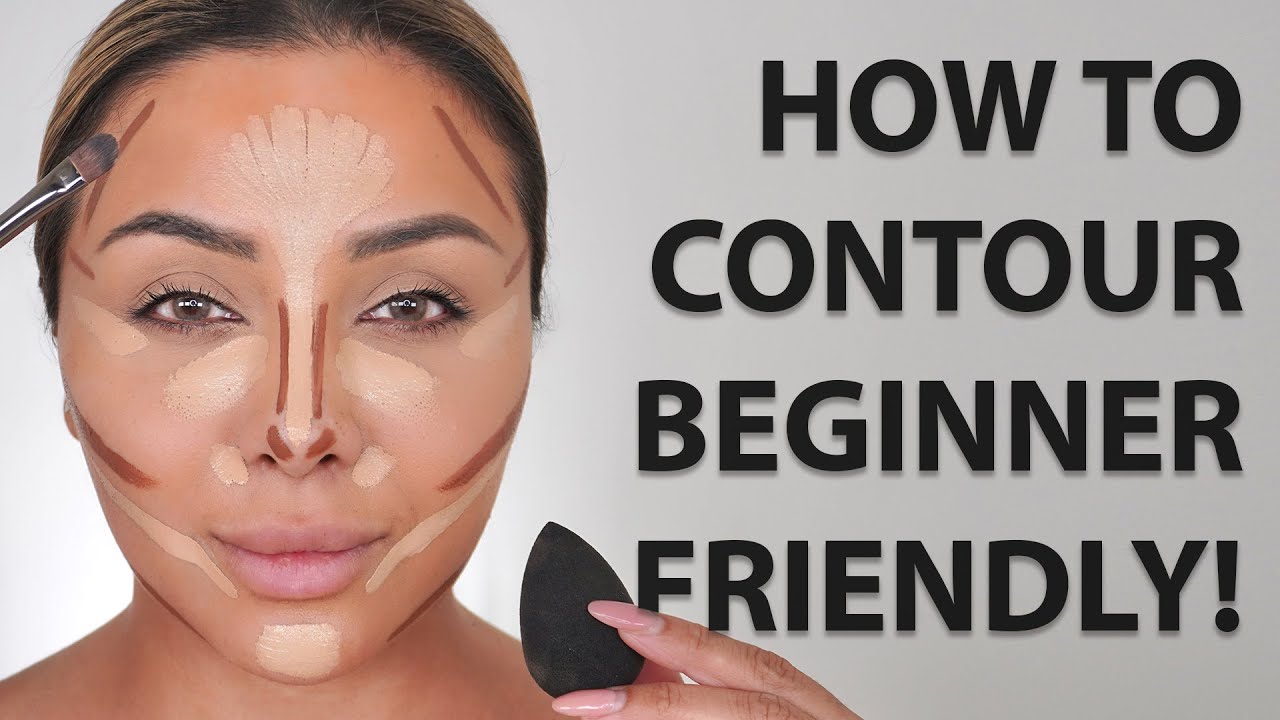This detailed advertisement image features a woman in the midst of contouring her face, with a clear demonstration of makeup application techniques aimed at beginners. The woman has brown and black hair, tied back to keep it out of her face. Her nails are painted pink, matching her pink lips, adding a touch of femininity to her appearance. She is holding a makeup applicator, possibly a sponge or a scraper that resembles a guitar pick, in her left hand. 

The woman's face is meticulously marked with contouring lines: darker brown shades are applied along the sides of her nose, below her cheeks, above her eyebrows, and on either side of her forehead. Lighter beige tones are blended across her forehead, down the center of her nose, below her eyes, along her cheekbones, around her mouth, and on her chin. 

A makeup brush is depicted touching her right forehead, indicating the ongoing application process. The backdrop is a plain gray, making the instructional text on the right side of the image stand out. The bold black text reads, "How to Contour: Beginner-Friendly!" emphasizing the instructional and accessible nature of the advertisement. 

This clear and detailed depiction highlights the steps involved in contouring, making it easy for novices to understand and replicate the technique.